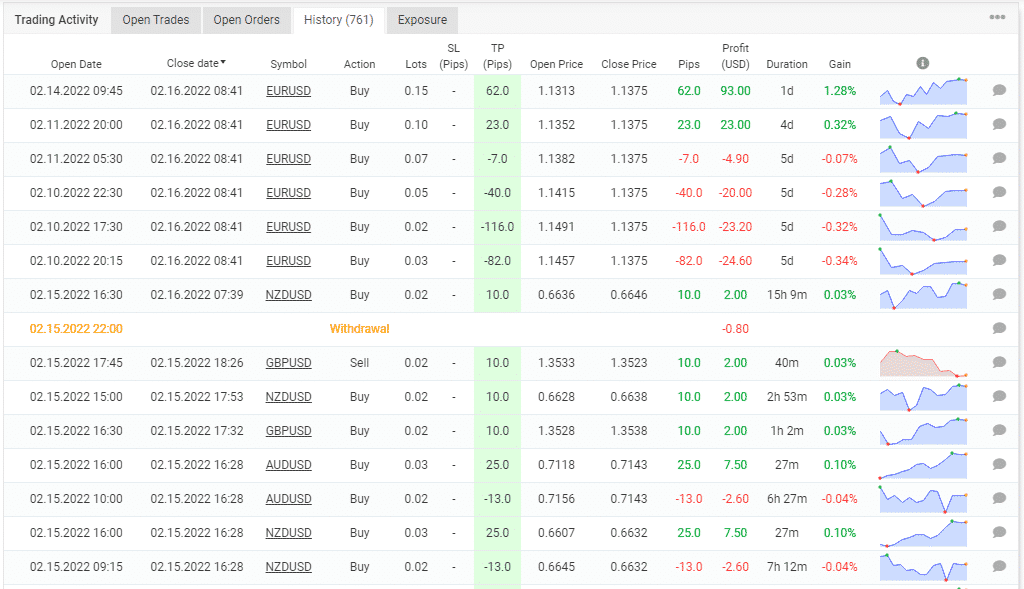The image displays a detailed table showcasing an individual's currency trading activity, specifically involving transactions from Euros to US Dollars. The table meticulously records various actions such as buying, specifying the quantities and corresponding prices. Accompanying the table are graphs that illustrate the entry and sale prices, providing a visual representation of these transactions. Additionally, a column is dedicated to the profits earned, along with a percentage gain column to highlight the performance metrics.

There are several tabs above the table, including Exposure, Open Orders, Open Trades, and Trading Activity, with the current tab labeled 'History' indicating a total of 761 rows of trading data. Notably, in the top right-hand corner of the interface, there are three small grey dots, commonly representing additional options or settings. One specific column includes an action labeled 'Withdraw' highlighted in orange, contrasting against the regular 'Buy' actions, which are in black.